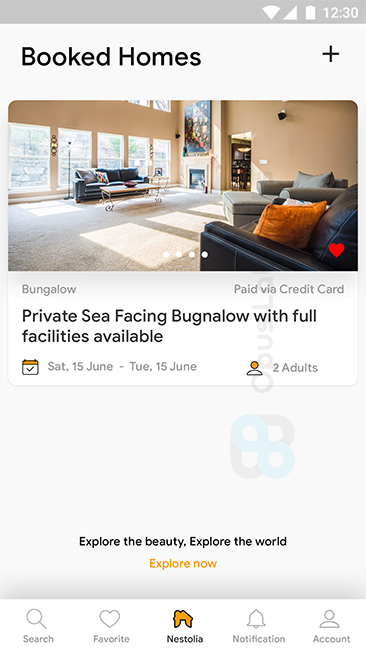Caption: 

The image features promotional material from "Booked Homes." Below the title, there is a photograph with its top two corners artistically rounded. The photograph showcases an expansive and airy room characterized by its minimalistic decor. Large, nearly wall-to-wall square windows line one side of the room, allowing for an abundance of natural light to flood the space. The high ceilings contribute to the room's open and airy feel. A notable feature within the room is a large piece of artwork hanging prominently. There is also a doorway leading into another room.

The center of the room is adorned with three beige rugs strategically placed on top of a larger brown rug, underlining the room's understated elegance. Sunlight either streams through skylights or from a side angle, enhancing the room's brightness.

Below the image, there is a description stating: "Bungalow: Private sea-facing bungalow with full facilities available. Booked from Saturday, June 15th to Tuesday, June 18th for two adults.” The tagline encourages exploration with the phrases: "Explore the beauty, explore the world, explore now."